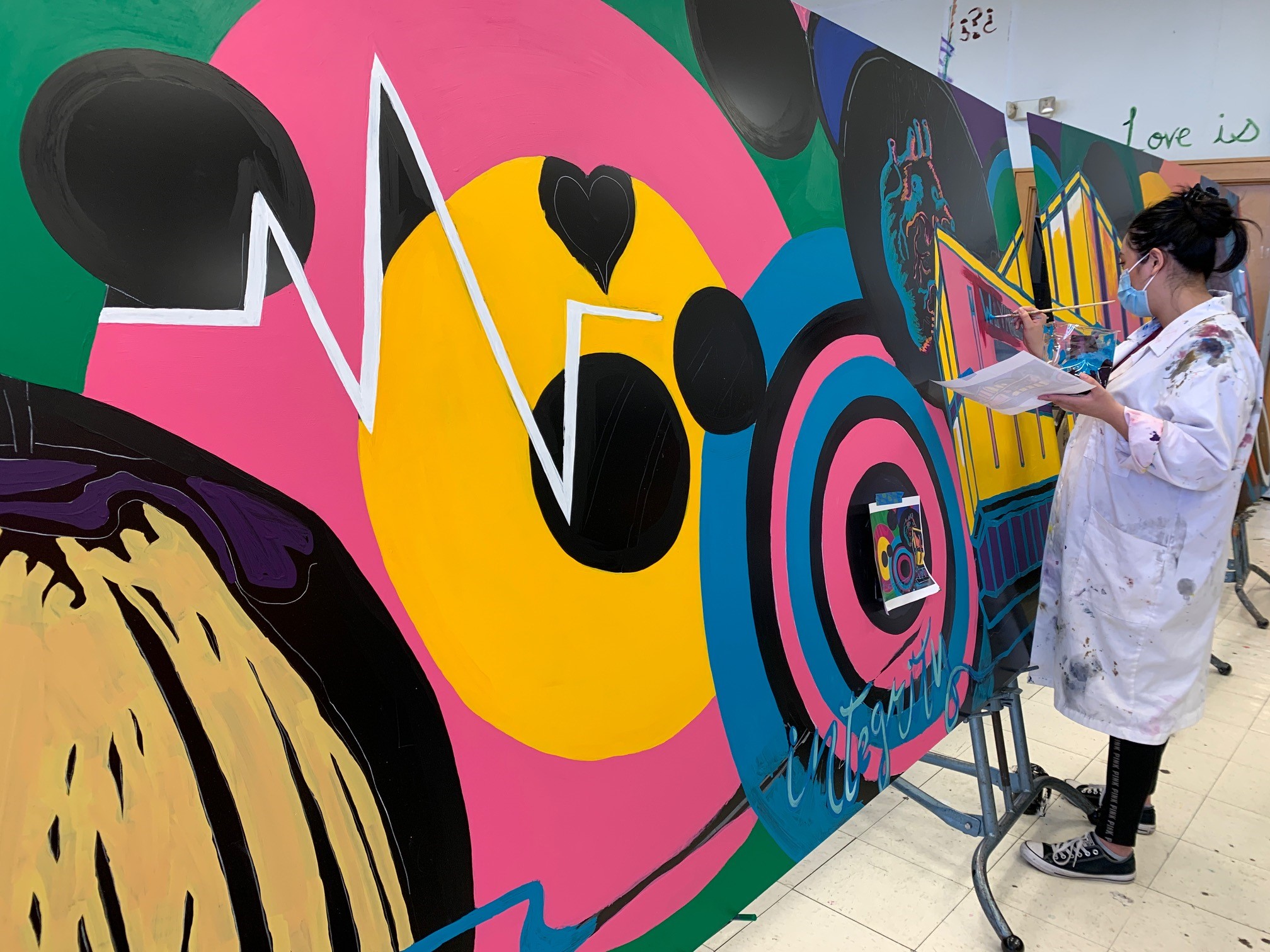In this image, we see a painter diligently working on a large, abstract mural that spans nearly the entire width of the backdrop. The floor beneath her is covered in pristine white tiles. She is positioned to the right side of the image, donned in a long white lab coat speckled with colorful paint splotches, black leggings, and black and white Converse shoes. Her black hair is pinned back neatly, and she is wearing a blue PPE face mask.

The mural appears to have an 80s inspired abstract design featuring a series of concentric circles in various colors—black, pink, yellow, and green—and a white heartbeat-like line running through them. An anatomical heart is painted towards the center, adding a unique touch to the composition. The painter holds a small piece of paper in her left hand, likely a reference image, while her right hand skillfully maneuvers a paintbrush.

Above this vibrant artwork, the words "love is" are written in green on the white wall, and near the bottom of the mural, the word "integrity" is inscribed in light blue cursive, overlapping several of the colorful circles. A smaller version of the completed mural is taped up in the center of the canvas, serving as a guide for the painter as she recreates the intricate design on this extensive wall space.